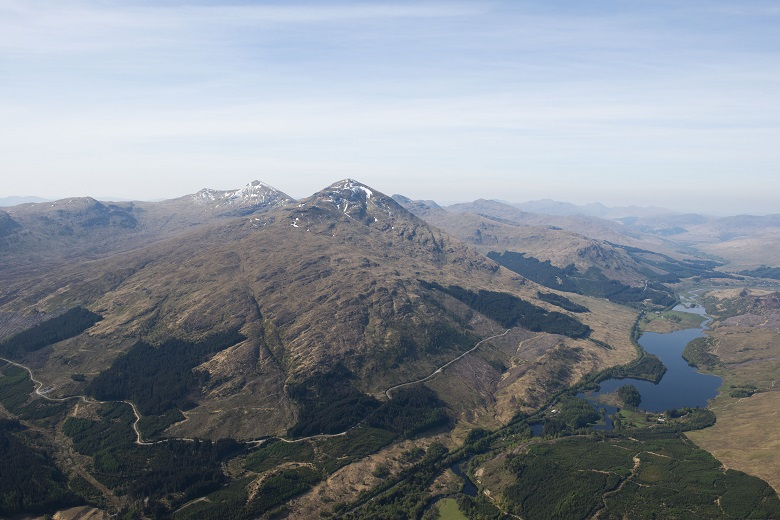The image captures a captivating mountain range, dominated by a central mountain with a broad, somewhat flat summit rather than a sharp peak, inclined at over a 45-degree angle. Snow delicately caps the central mountain and the adjacent one to its left, standing out as the only snowy features. Beyond this, the image showcases a few smaller peaks, predominantly on the left side, with sparse peaks on the right.

The upper third of the photo is dominated by a serene blue sky streaked with lighter blue hues. As the eye moves downwards, the mountains transition from a distant purple hue to a closer brown, reflecting the varied terrain. Green areas emerge prominently around the base, accentuated by clusters of trees and greenery particularly vibrant near a body of water on the right. This water source appears to be a lake, feeding into a small river that meanders from it.

At the base of the mountains, the landscape is dotted with roads winding from left to right, and the bottom right corner harbors a dense cluster of lush trees. The green surrounding the lake contrasts sharply with the predominantly brown landscape, adding depth to the overall scenery. The sky remains mostly clear with a few scattered clouds, contributing to the tranquil vista.